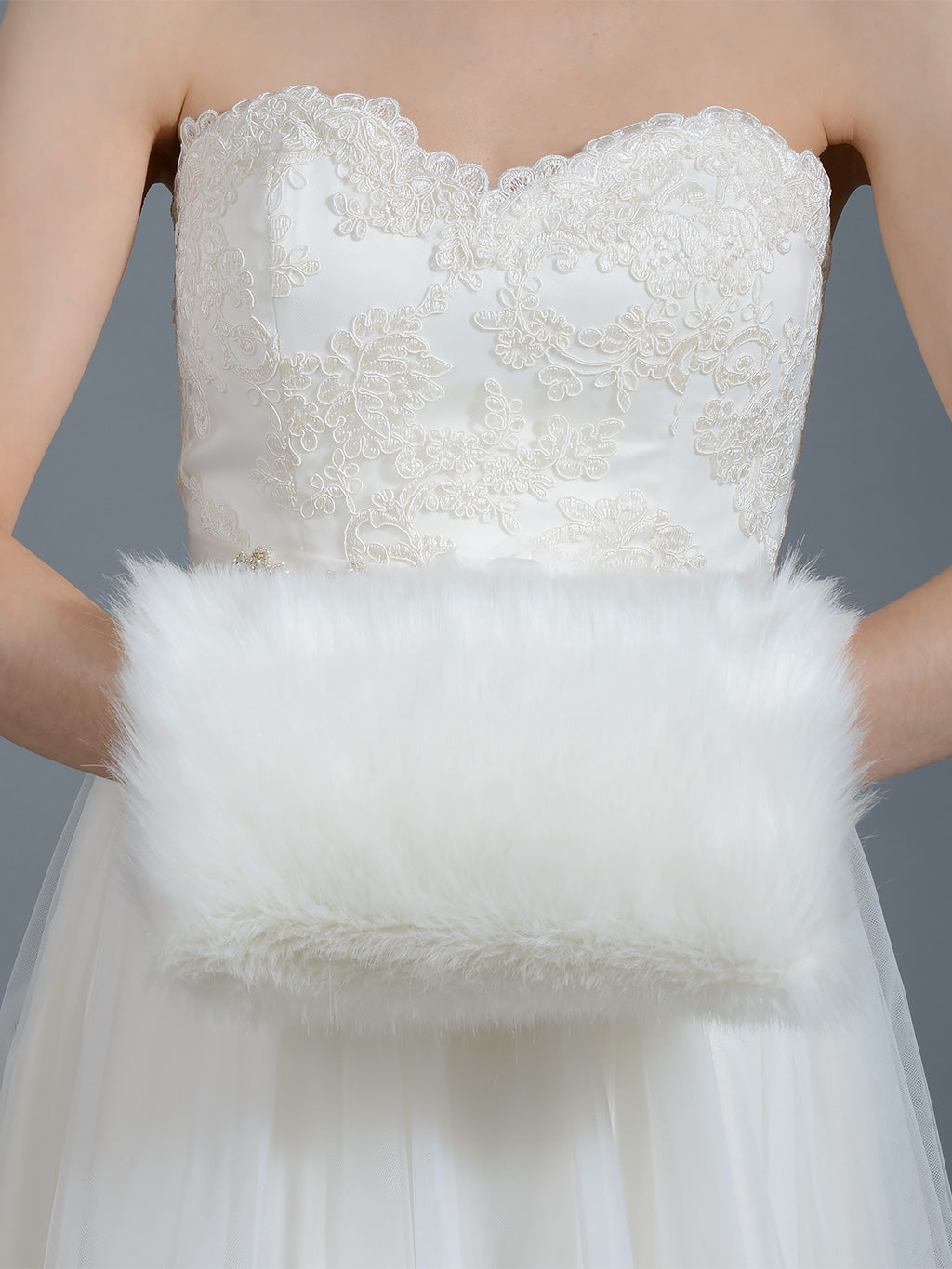The image showcases a woman with light skin, dressed in a strapless, sleeveless wedding gown, visible from the shoulders to mid-thigh. The wedding dress has a sweetheart neckline, with intricate lace appliqué adorning the bodice, and the skirt features a delicate tulle overlay. Her arms are gracefully bent in front of her, held inside a cylindrical, fluffy white fur muff, which adds a touch of elegance and warmth to her ensemble. The background is a serene light blue, providing a simple yet complementary contrast to the white dress and muff. Overall, the details and colors in the photo—white, light flesh tones, and the light blue background—accentuate the bridal theme, possibly highlighting the muff as a unique accessory for a winter wedding.